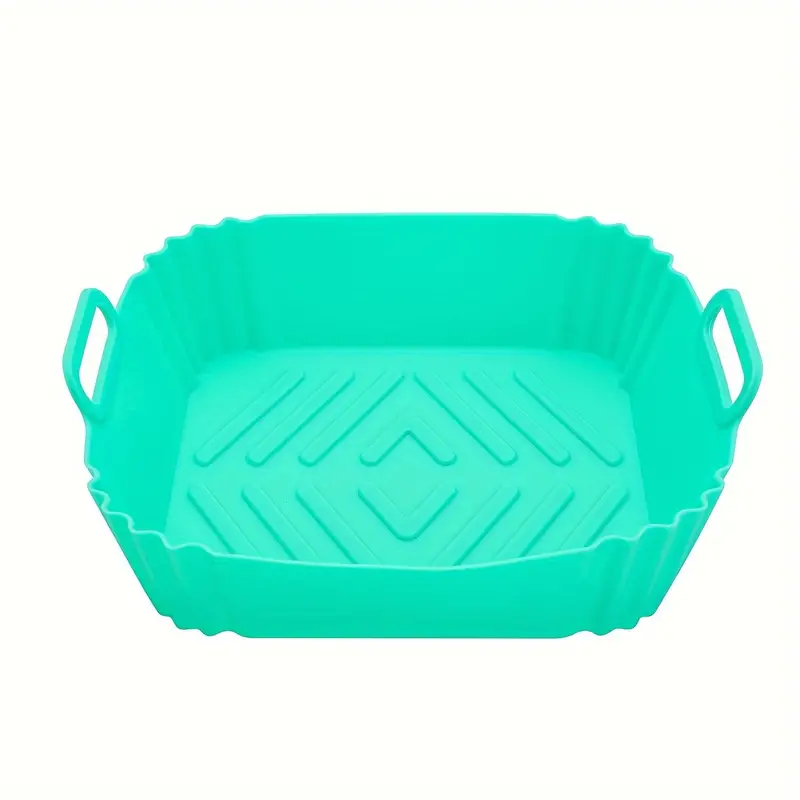This image features a large, rectangular, teal-colored plastic container that appears versatile enough for various uses such as organization or storage. Measuring approximately 2 by 3 feet with a depth of about 12 inches, the container’s substantial size and robust build suggest it could hold a significant amount of items, be it laundry, baking supplies, or other household goods. The container is made of thick, molded plastic with smoothly curved corners and integrated handles on its shorter ends for easy carrying. The bottom surface of the container is designed with grooves or a 3D texture, likely to provide traction and prevent slipping, while potentially aiding in the separation of items stored within. The overall structure, including the slightly expandable corners, emphasizes its durability and heavy-duty capacity. The background of the image is stark white, highlighting the container's turquoise hue and detailed features.